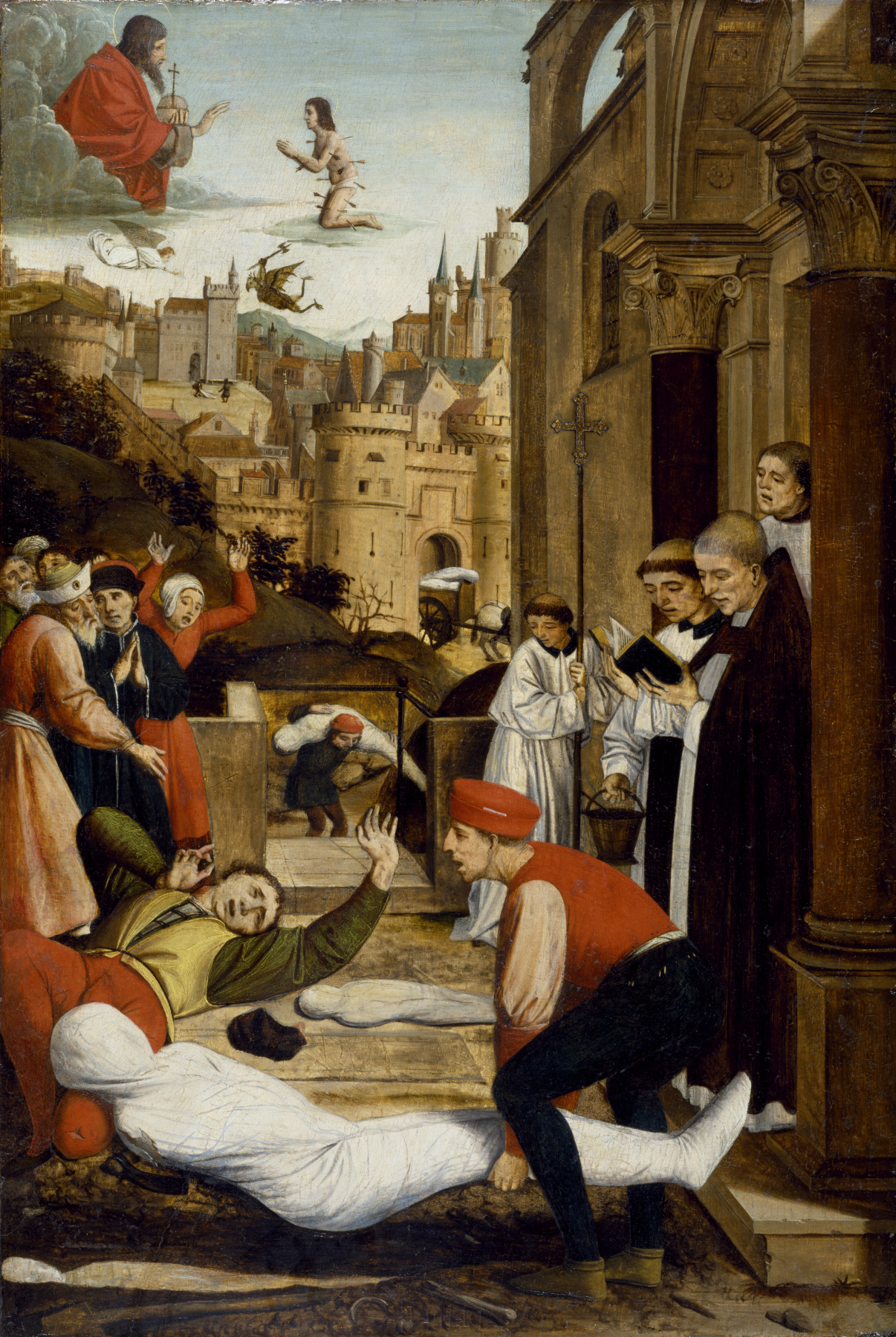The detailed image depicts an old religious painting set in a historical cityscape, likely from the Renaissance or earlier centuries. On the right, a priest and clergymen, dressed in white robes with distinctive tonsured haircuts, are reading from an open Bible. Surrounding them are church attendants, some carrying bodies wrapped in white linen, resembling mummies. One man in orange pants and a yellow vest, with an olive-green long sleeve underneath, is seen in distress on the ground with outstretched arms. Another figure is lifting a wrapped corpse. 

In the background, tall buildings resembling castles and towers add depth, while the sky features a dramatic biblical scene. Jesus, cloaked in a red robe, emerges from the clouds holding a cross. Kneeling before Him is a nearly naked person, pierced by multiple arrows, hands clasped in desperate prayer. Above them, an angelic or demonic figure with wings appears to be wielding a sword, adding to the painting's dramatic tension. Women and other onlookers on the ground exhibit expressions of anguish and despair, their hands raised as if pleading or mourning amidst an atmosphere suggestive of a great plague or a divine intervention.